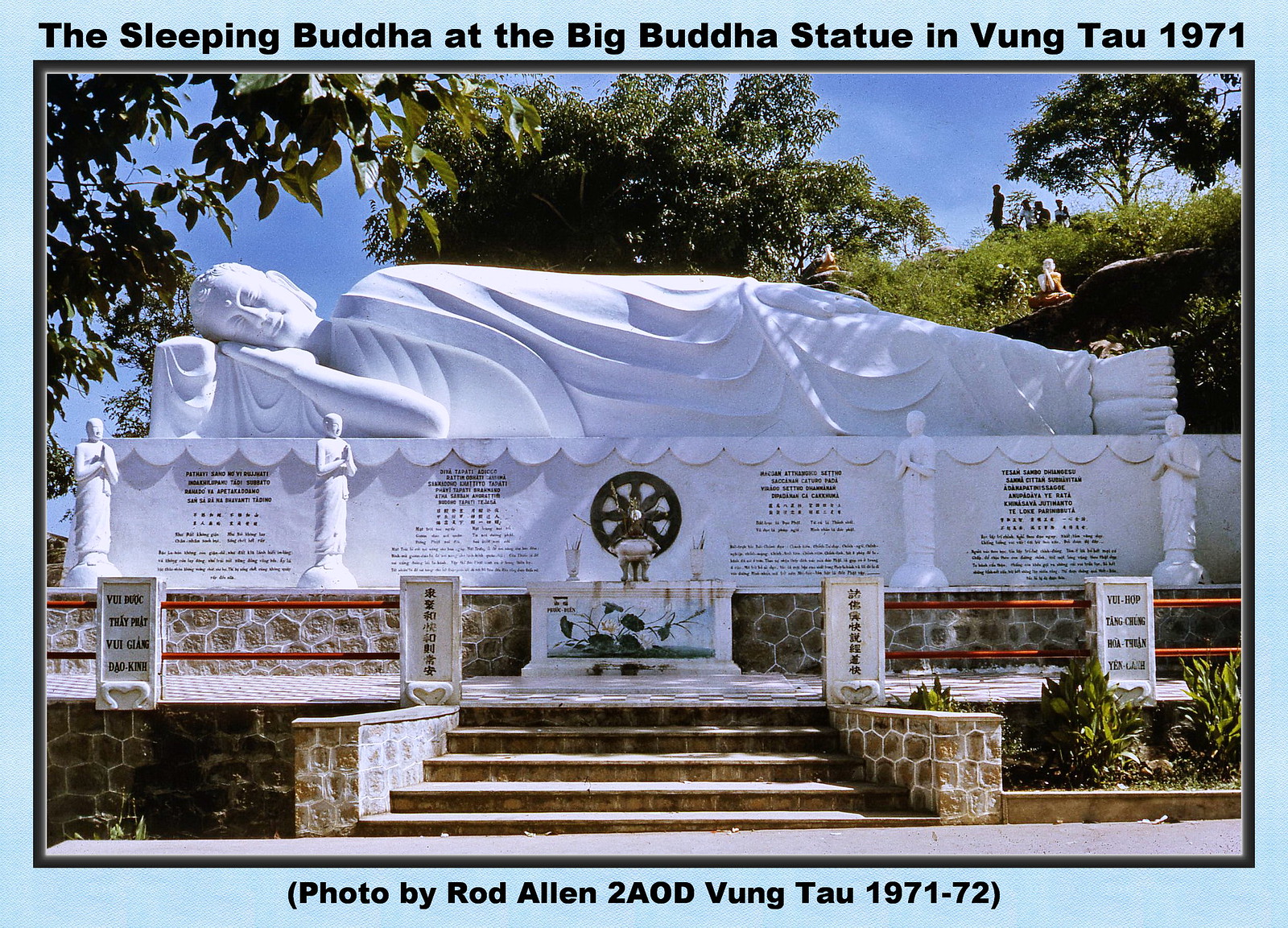This image, taken during the Vietnam War, is a clear, well-composed photograph captured by Rod Allen from the 2nd Australian Ordnance Depot (2AOD), Vung Tau, between 1971 and 1972. Depicting the Sleeping Buddha at the Big Buddha Statue in Vung Tau, the photo showcases a large white statue of the Sleeping Buddha lying on its side in a serene valley with lush greenery and significant tree presence. In front of the Buddha are four smaller statues, likely Buddhas or praying monks, positioned before a staircase leading to an upper platform. The scene is set during the daytime, possibly early evening, as suggested by the lighting and shadows. People are seen atop a hill behind the main statue, adding depth to the landscape. The pedestal of the Sleeping Buddha is adorned with black text in various languages, providing context to this tranquil, historical setting.